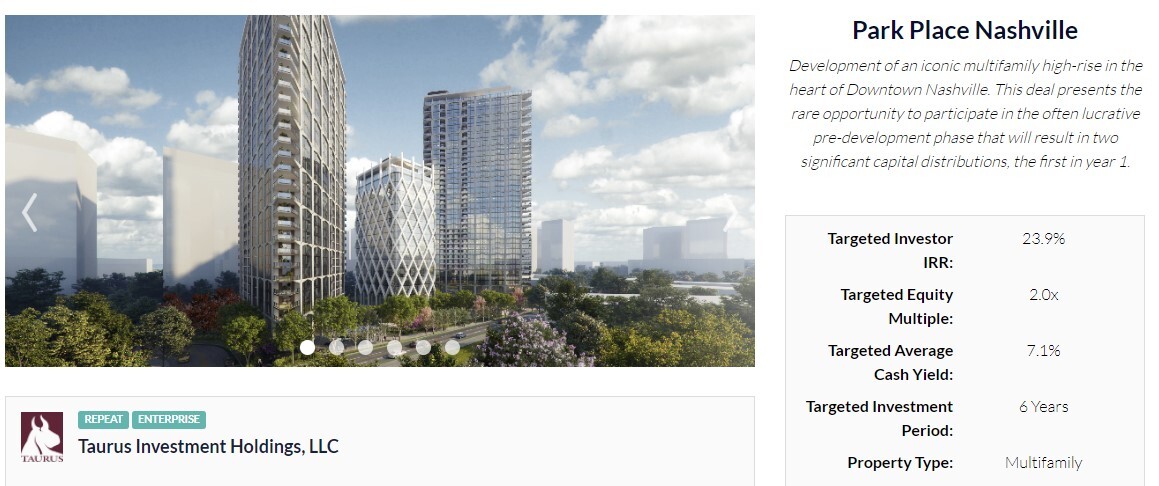The left side of the image shows a picturesque area enclosed within a square, featuring tall, sleek silver and gray buildings under a serene blue sky dotted with white clouds. At the base of these buildings, there is lush green shrubbery and trees, adding a touch of nature to the urban scene. Below the image of the buildings, the text "Taurus Investment Holdings, LLC" is visible. Above this text, set within a green rectangle, is the word "Enterprise," and to its left, the word "Repeat." 

On the right side of the image, the text reads "Park Place, Nashville," followed by a brief description stating, "Development of an iconic multifamily high-rise in the heart of downtown Nashville. The deal represents the rare opportunity to participate in the often lucrative pre-development phase that will result in two significant capital distributions, the first in year one."

To the left, within another square running vertically, there are key investment metrics listed: "Targeted Investor IRR," "Targeted Equity Multiple," "Targeted Average Cash Yield," "Targeted Investment Period," and "Property Type." To the right of these metrics, the corresponding figures are listed as follows: 23.9%, 2.0x, 7.1%, 6 years, and "Multifamily."